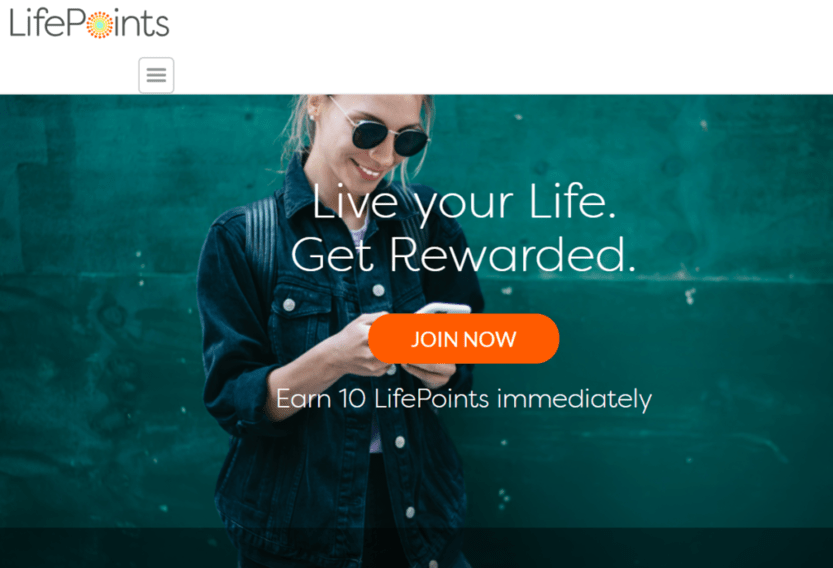This is a screenshot of the Life Points app or website. In the top left corner, you can see the Life Points logo, where the 'O' in 'points' is depicted as a geometric shape filled with colorful dots. Below the logo, there is a small drop-down menu. 

The main focus of the page is a large background image of a woman smiling as she looks at her phone. She is wearing black glasses, a black denim jacket, a light-colored top underneath, and possibly black pants. The wall behind her is a dark emerald color, adding a rich backdrop to the scene. 

Overlaying this image is text that reads, "Live your life, get rewarded." Beneath this text, there is an orange button with white text that says, "Join Me." Directly below the button, additional white text reads, "Earn 10 Life Points immediately."